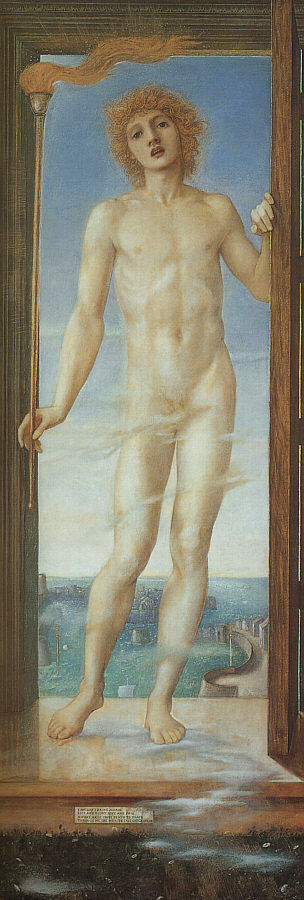The painting depicts a nude male figure with pale skin standing inside a long, narrow frame that resembles a window. He has curly, reddish-blonde hair that forms a halo around his head, reaching down to his shoulders. In his right hand, he holds a long, golden rod with a wispy flame emanating from it, resembling a torch. His left hand is placed against the frame, and he leans slightly to the right. The man's build is trim, not overly muscular but in good shape. Wispy clouds strategically obscure his crotch, adding a modest touch to the artwork. Behind him, there is a body of water with hints of buildings or a bridge in the background, topped by a blue sky. His open mouth adds a dynamic element to his serene yet powerful stance.